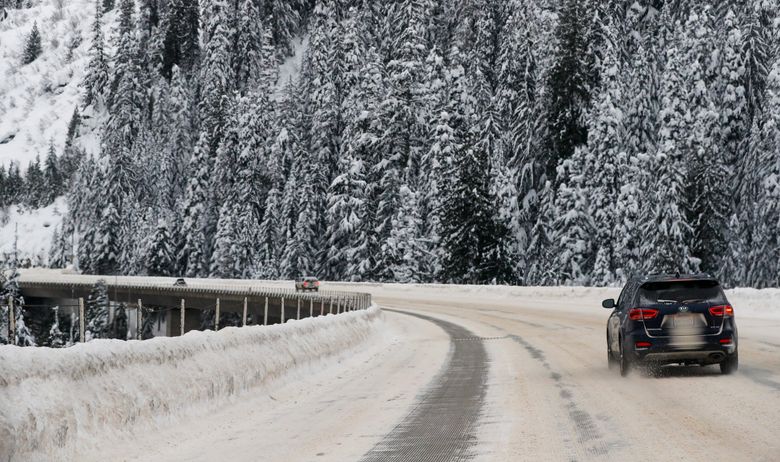The photograph captures a serene, wintry scene of a roadway carved into a mountainside, flanked by a dense, snow-laden evergreen forest. The road, partially plowed with snow piled up on either side, reveals only two visible vehicles. In the foreground, a dark SUV with red taillights leaves tire tracks as it moves away from the viewpoint, hinting at possibly slippery conditions. In the distant background, a small red vehicle travels in the opposite direction on what appears to be an elevated bridge overpass. Tall trees, heavily laden with snow, form a majestic, dense backdrop, enhancing the tranquil, wintry atmosphere.